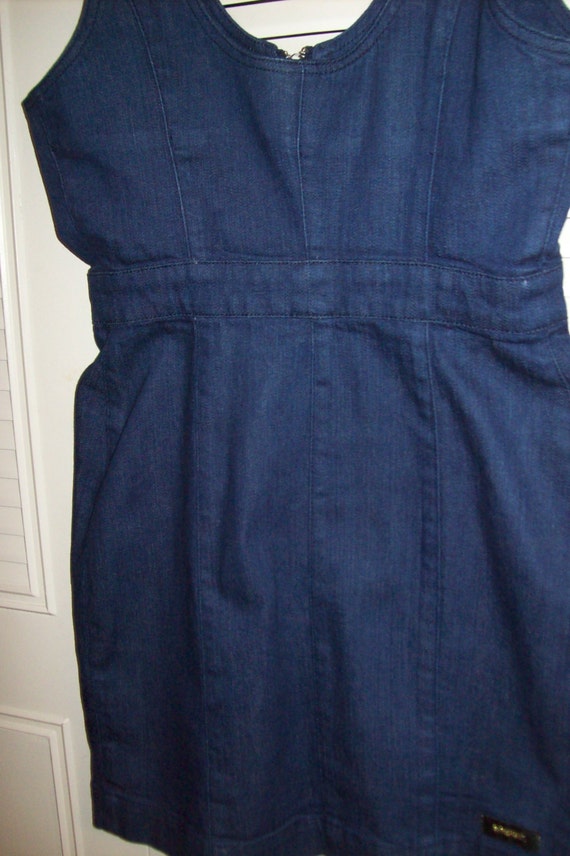The image features a blue, sleeveless denim dress hanging from the top of a white louvered closet door. The dress, appearing to be of women's style, has a zipper running down the back and a label that is not easily readable but suggests it is a branded garment. The fabric displays a deep, true denim color with visible folds and seams—two on one side and one down the middle. The dress has a mid-chest cinch and an empire waist adorned with a one to two-inch thick belt. This photograph, which appears to be taken vertically by a human, captures a simple, handmade-looking yet branded piece of clothing against a non-professional setup, including a white wall or closed blinders in the background.